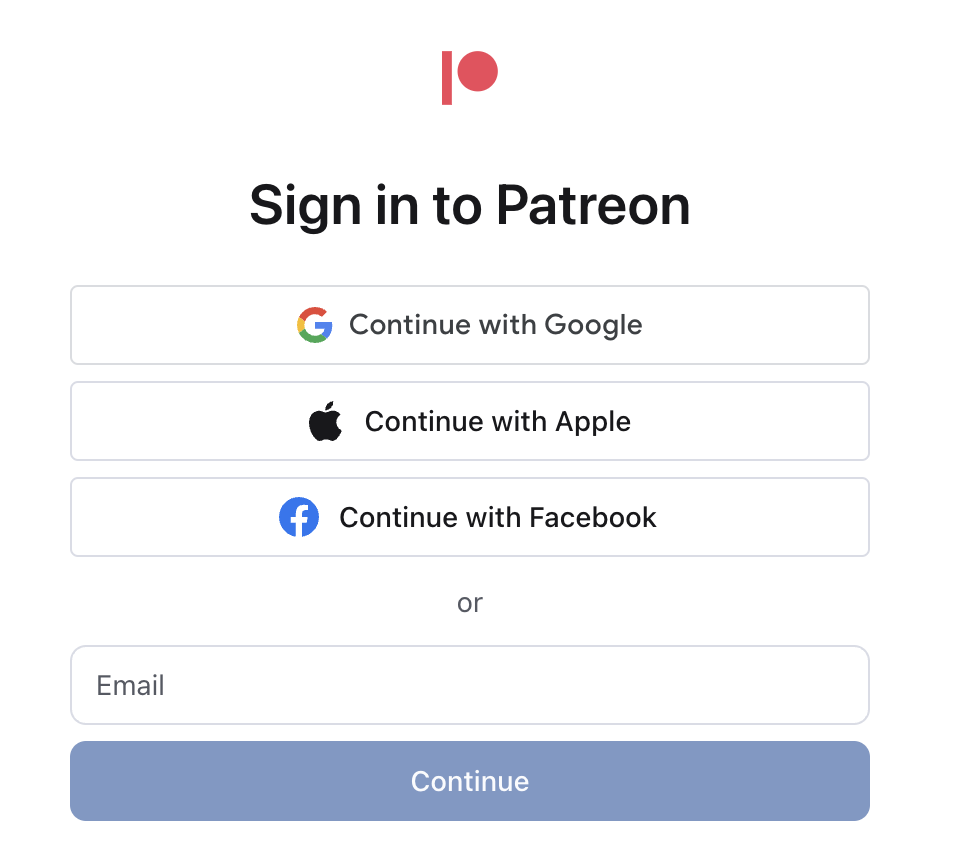The image displays the login interface for Patreon with a sleek and minimalistic design against a completely white background. At the top center is the recognizable Patreon symbol, a vertical red rectangle adjacent to a red circle, forming a stylized 'P.' 

Directly beneath the icon, the title "Sign in to Patreon" is prominently displayed in black font. Below the title are three distinct buttons for alternative sign-in options: the first features the Google icon with the text "Continue with Google," the second showcases the Apple icon alongside "Continue with Apple," and the third presents the Facebook icon paired with "Continue with Facebook." All three buttons use black text and are outlined in a bluish-gray color.

Further down the interface, the word "OR" in black provides an alternative option to sign in using an email address. Below this, a text box allows users to input their email, maintaining the same bluish-gray outline as the previous buttons. 

At the very bottom of the image, there is a bluish-gray colored button with the word "Continue" in white font, standing out as the final actionable step for users to proceed with their login. Overall, the color scheme and layout prioritize clarity and ease of use.